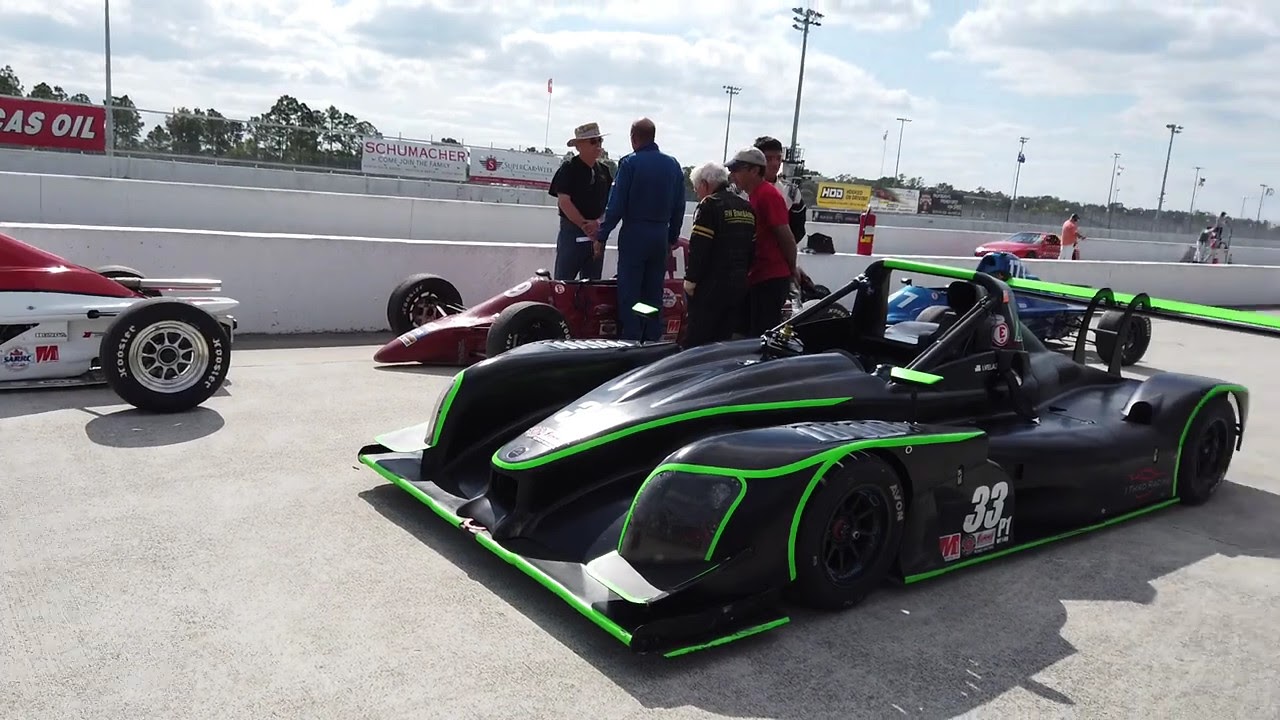The image depicts a vibrant scene at an outdoor racetrack under a blue sky with puffy white clouds. At the center of the photograph, five men are engaged in conversation, gathered around a red race car with a sharp nose. Surrounding them are various race cars positioned on the cement track. To the left of the image, partially visible, is a race car that is red on top and white on the bottom. Dominating the foreground is a black car with neon green accents, bearing the number 33 in white on its side door. This car stands out with its matte finish and distinctive green detailing, notably on the spoiler and front bumper. In the background, additional men, signs on the fence, and tall poles with streetlights add to the bustling atmosphere of the raceway, enhancing the dynamic and lively setting of the racetrack.